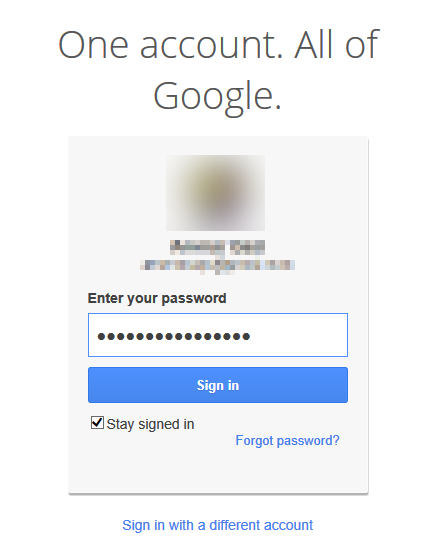This image appears to be a screenshot from a mobile device displaying a Google sign-in page. At the top, there's a heading in bold text saying "One account. All of Google." Below this text, there is an icon representing a Google app, but the app name and icon are blurred out and obscured. 

The main part of the image shows a prompt to "Enter your password," followed by a password input field filled with approximately 14 black dots, indicating hidden characters. Directly beneath this, there is a blue "Sign in" button. Additionally, there is an option with a checked checkbox labeled "Stay signed in" and a hyperlink text in blue that reads "Forgot password."

A gray horizontal line separates these elements from the final portion of the image, where there's another blue hyperlink text that says "Sign in with a different account." The rest of the screen is primarily white space, adding to the simplicity and focus of the sign-in interface. The reason for the blurring of the app icon and name is unclear.